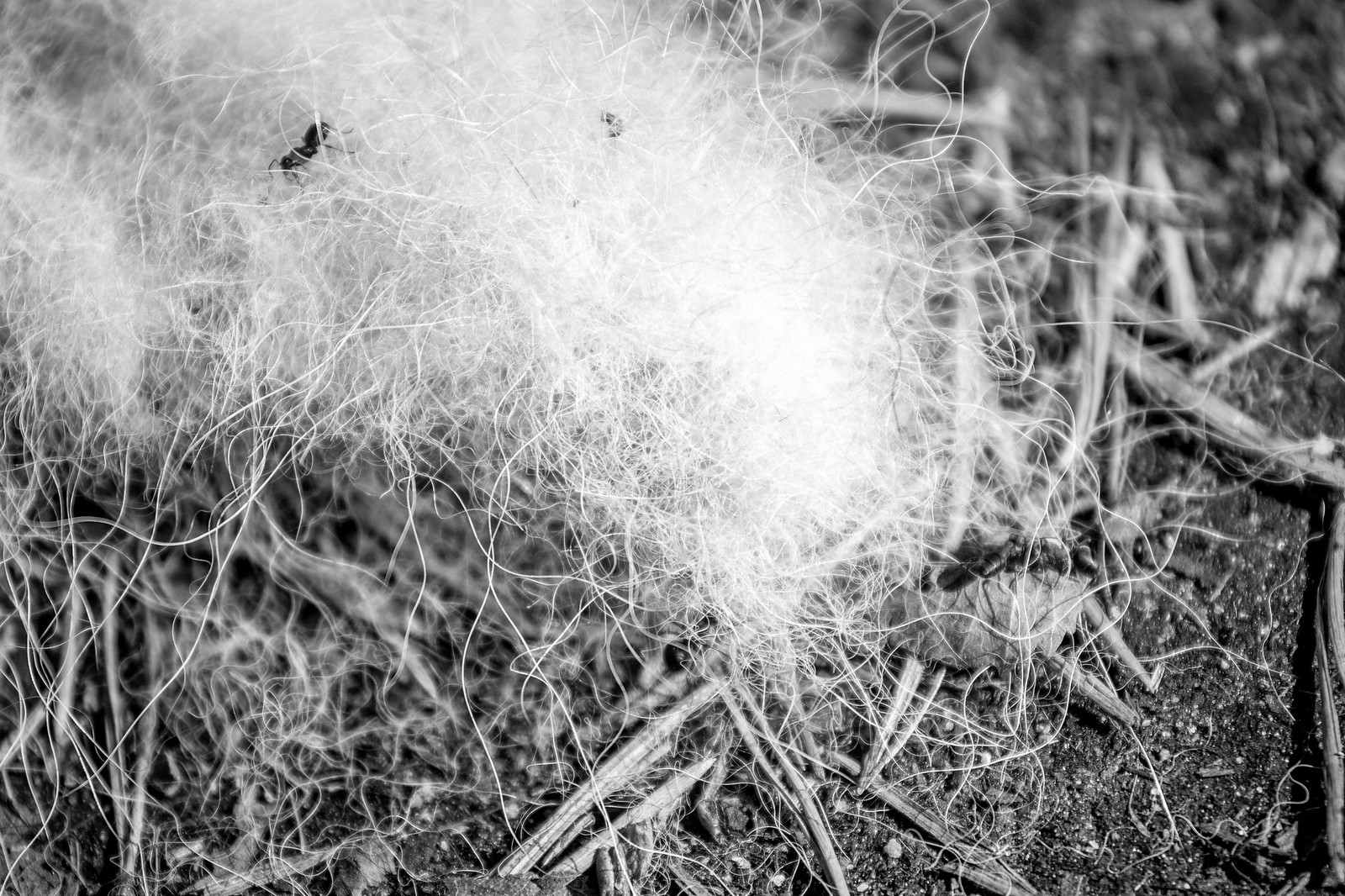The black and white photograph depicts a perplexing scene of what appears to be a chaotic, dense clump of white, wiry material concentrated in the upper left and spreading outwards. The material, which could be plant fibers, the stuffing from a cushion, or even shorn wool, forms a thick, cotton-like, and stringy mass. Within this tangled, cloud-like structure, two small, dark insects—possibly ants—are trapped, their black bodies starkly contrasting against the white fibers. The bottom layer of the image shows the ground covered with dirt and scattered, dead vegetation such as limbs, grass, and weeds. The overall impression is one of disarray and entrapment, as nature's remnants coexist with the mysterious, fibrous cluster.